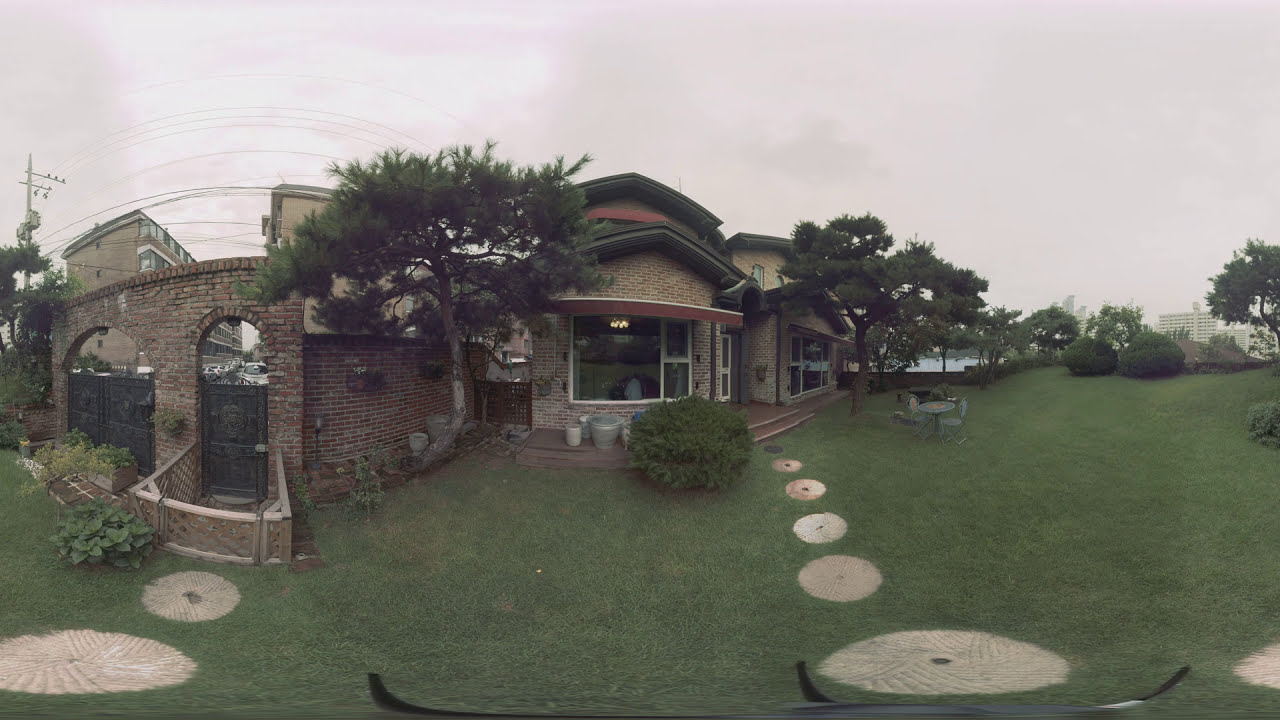The image depicts a lush, green yard in front of a two-story brick house. The yard features a circular footpath composed of pavers or circular objects, leading toward the house. Several green bushes and trees surround the house, and additional foliage and a tall, white building are visible in the background. The house itself prominently displays a large window on the front and right side, and a door with a large gate on the left. Power lines and a power pole are seen running above the house. Inside, there are visible lights, suggesting that it’s daytime despite the cloudy, overcast sky. In the distance, other houses and skyscrapers suggest the house is situated in a relatively urban environment possibly near water, as there are hints of a lake or ocean in the background. The yard also contains a circular lawn table and chairs, enhancing the inviting outdoor setting.